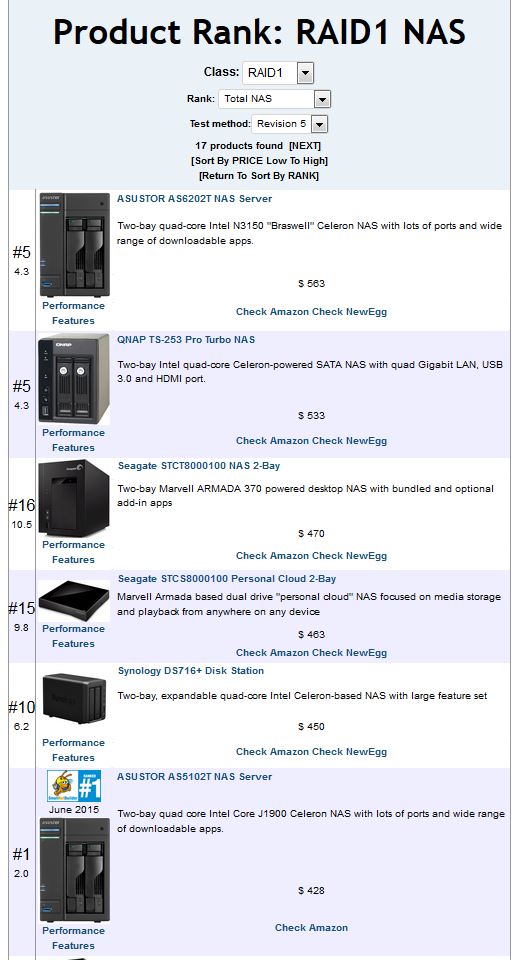Screenshot titled "Product Rank RAID 1 NAS"

This screenshot features detailed rankings and specifications for various RAID 1 NAS products. Three drop-down windows are displayed: 

1. **Class**: Set to "RAID 1".
2. **Rank**: Set to "Total NAS".
3. **Test Method**: Set to "Revision 5".

Below these drop-downs, the interface indicates that 17 products have been found. A list of these computer accessories follows, each including a number, a star rating, the name, and an image of the product.

### Product Listings:

1. **ASUStor AS6202T NAS Server**
   - **Description**: A sleek black-cased NAS server featuring a 2-bay, quad-core Intel N3150 Braswell Celeron processor.
   - **Features**: Numerous ports and a wide range of downloadable apps.
   - **Price**: $563
   - **Ratings**: Star rating of 4.3, ranked at number 5.
   - **Purchase Links**: Options to check prices on Amazon and Newegg.

2. **QNAP TS-253 Pro Turbo NAS**
   - **Description**: A robust 2-bay NAS with an Intel quad-core Celeron processor.
   - **Features**: Equipped with quad gigabit LAN, USB 3.0, and an HDMI port.
   - **Price**: $533

3. **ASUStor AS5102T NAS Server**
   - **Description**: Another high-quality NAS server by ASUStor, marked with a number 1 customer award.
   - **Price**: $428 

This detailed list is aimed at providing a comprehensive overview of leading RAID 1 NAS products, complete with essential information for making an informed purchase decision.